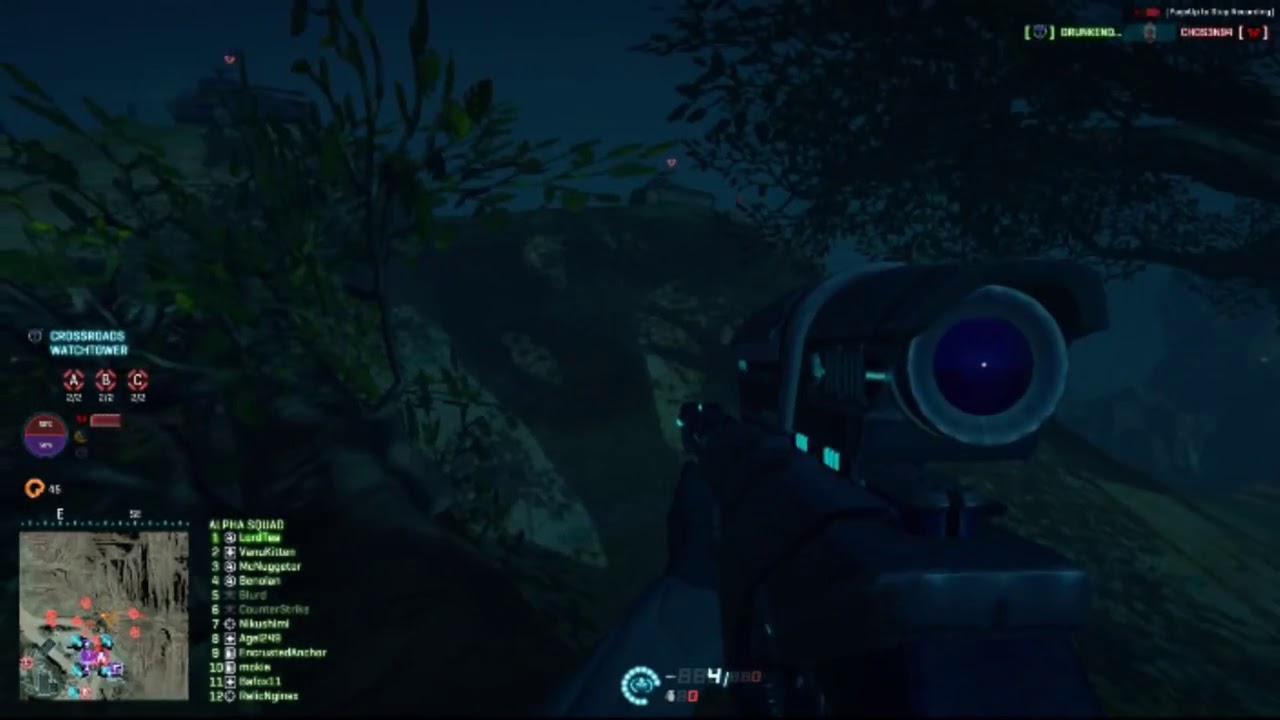This screenshot appears to be from a nighttime scene in a first-person shooter video game, characterized by a dark bluish hue. Dominating the foreground is a weapon held by a hand, visible through a blue sight. The background reveals a forested setting with numerous trees and vegetation spread across a sloped green hill under a dark sky, possibly illuminated by two faint red moons. To the left, light teal text indicates locations named "Crossroads" and "Watchtower," accompanied by icons labeled A, B, and C with red diamond outlines. Below each icon, white numbers are displayed: 270 under A, 212 under B, and 202 under C. Additional elements include a circular shape split into red and purple halves, each containing a white icon. The lower left corner features an area map with red dots and teal X's, likely indicating positions of players or objectives, and in green text, it shows "PHX Squad" followed by a list from 1 to 12, including several usernames. Other cluttered and largely unreadable texts and icons are scattered around the image, adding to the game's detailed HUD (Heads-Up Display).